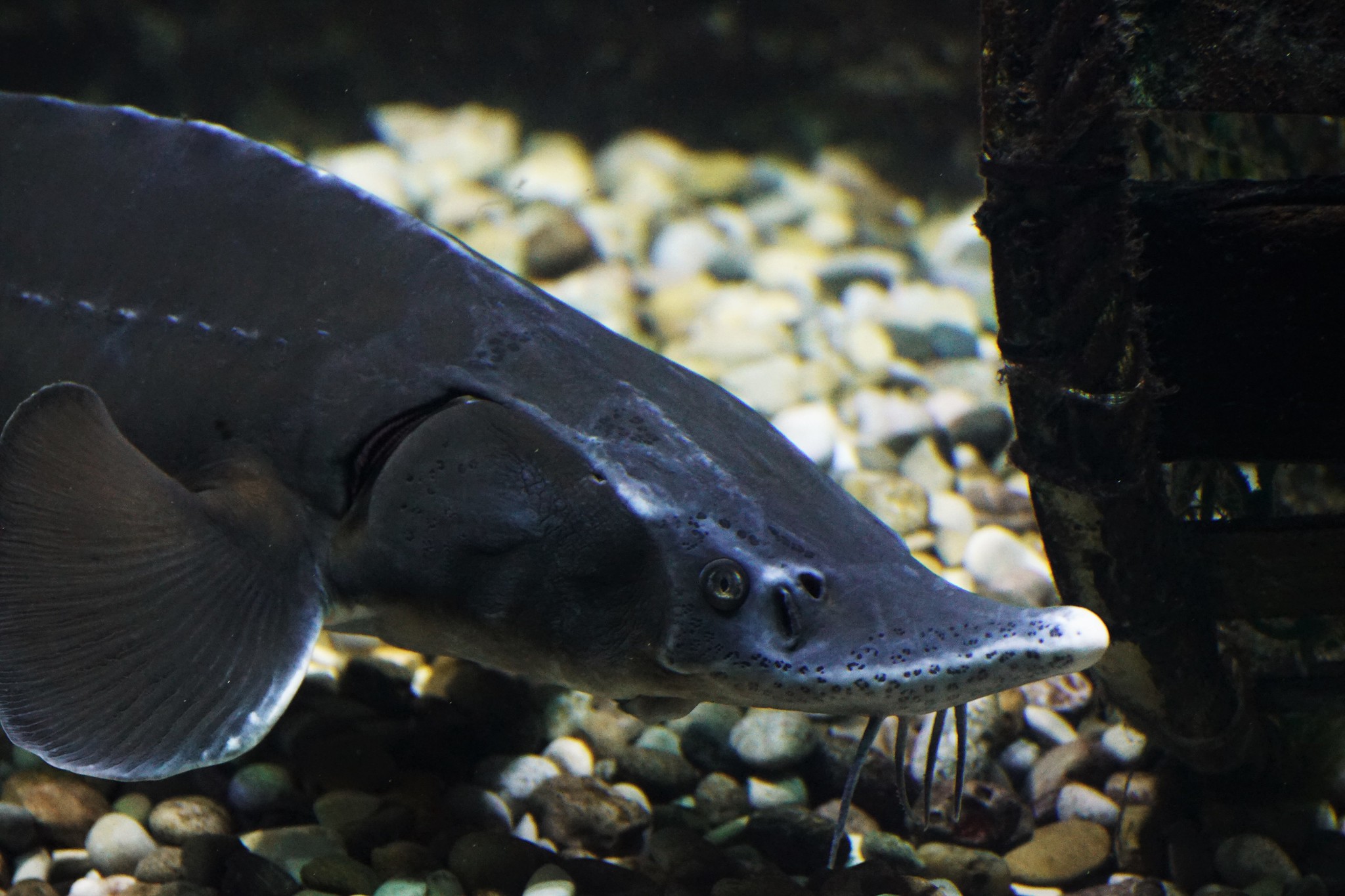The image is a horizontally rectangular, close-up photograph of a dark grey fish, possibly in an aquarium setting. The fish has a distinctive white bill-like mouth that slopes outward, reminiscent of a duck bill. Four skin-like appendages hang from its chin. Its body tapers to the left, and a seashell-shaped fin is visible. The background features a mix of gravel pebbles in shades of white, beige, yellow, brown, and black. On the right side, there is an indistinct dark object, possibly a rock structure or aquarium decor. The overall scene gives the impression of an underwater environment, although the presence of water isn't explicitly clear.